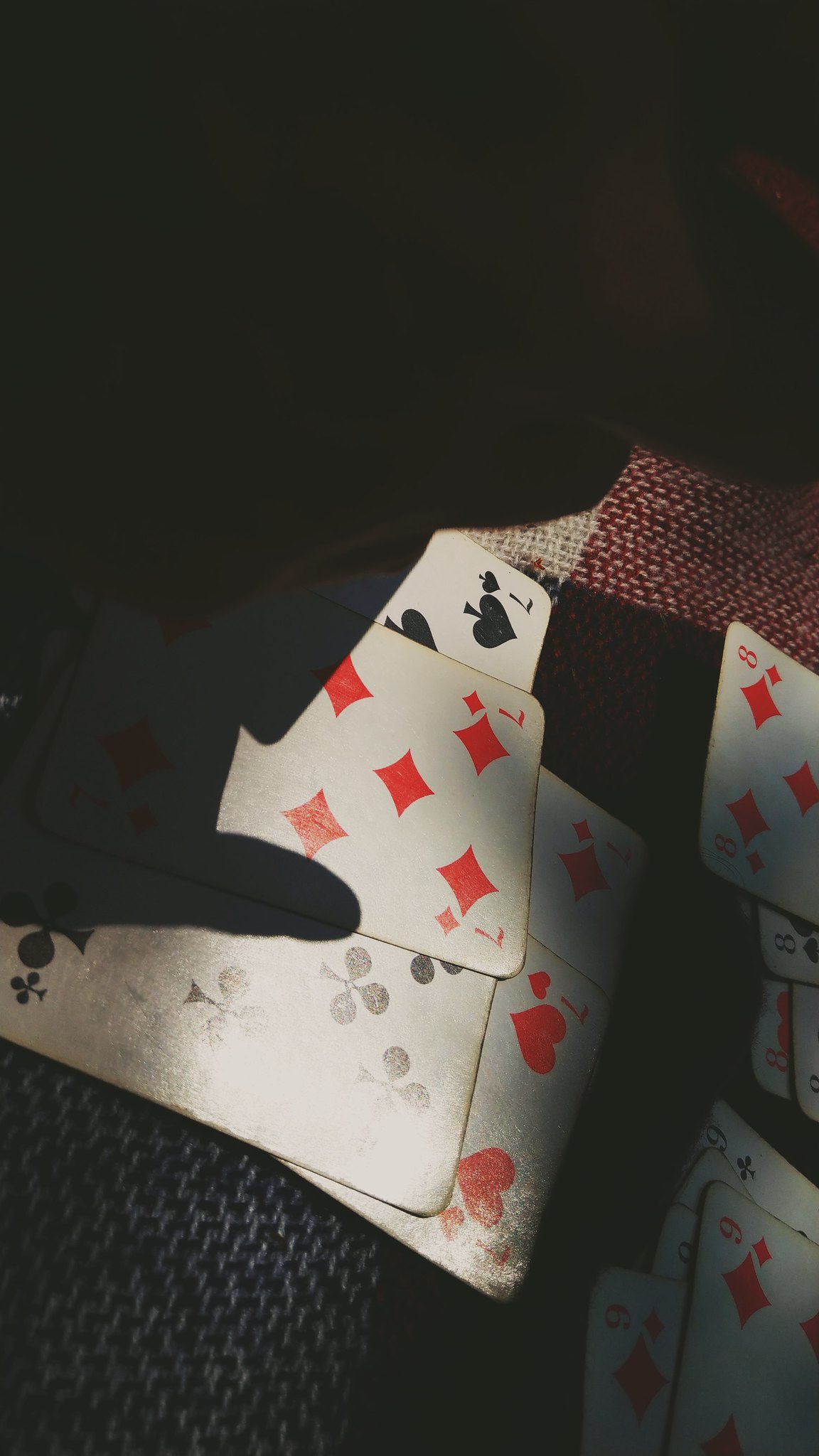In this dark and mysterious photograph, the scene appears cloaked in shadows, revealing just fragments of the setting. On the left, the faint outline of a left hand along with its thumb is barely visible against the blackness. This hand is positioned amidst a spread of playing cards laid out on what seems to be a gray placemat, likely resting on a table. Next to this gray placemat, there are two additional placemats: one tan-colored and the other with a reddish-yellow hue.

The series of playing cards displayed are slightly faded but discernible. Among them are a seven of spades, a seven of diamonds, a seven of hearts, and a partially visible card with a diamond suit. There are a total of five cards in this hand. In contrast, on the opposite side of the image, another hand is visible holding cards in various suits including diamonds, spades, and clovers. On the top right section of the image, more cards can be observed, including the eight of diamonds, the eight of spades, the eight of hearts, and an indistinct card. Despite the dimness, the image prominently features the subtle interactions and haphazard arrangement of the playing cards.